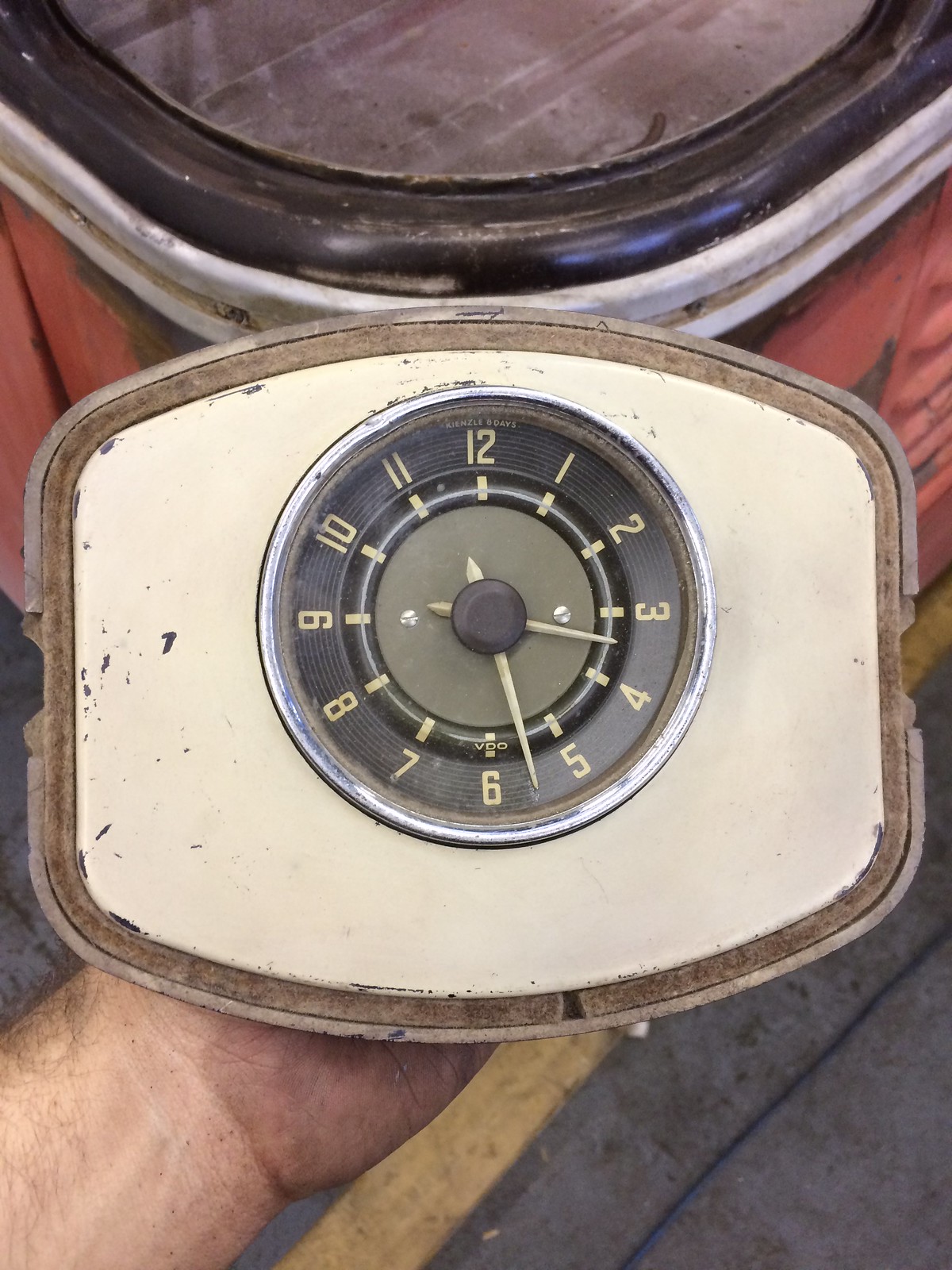In this vertically-oriented rectangular photograph, the viewer's gaze is drawn to a close-up of a hand, emerging from the lower left corner, holding an antique, beige-colored clock. The clock, reminiscent of ones found in vintage cars or boats, features a rectangular shape with rounded edges on the top and bottom. Central to the beige casing is a dark brown clock face adorned with tan letters or numbers marking the hours from 1 to 12. The clock reads 3:27, with its cream-colored hour and minute hands adding to its vintage charm. The piece appears aged, framed by a dark wooden rim that shows signs of deterioration and rot. Beneath the clock is a partially visible dark red table, possibly wooden, with a slatted design akin to a picnic table, enhancing the nostalgic feel of the scene.